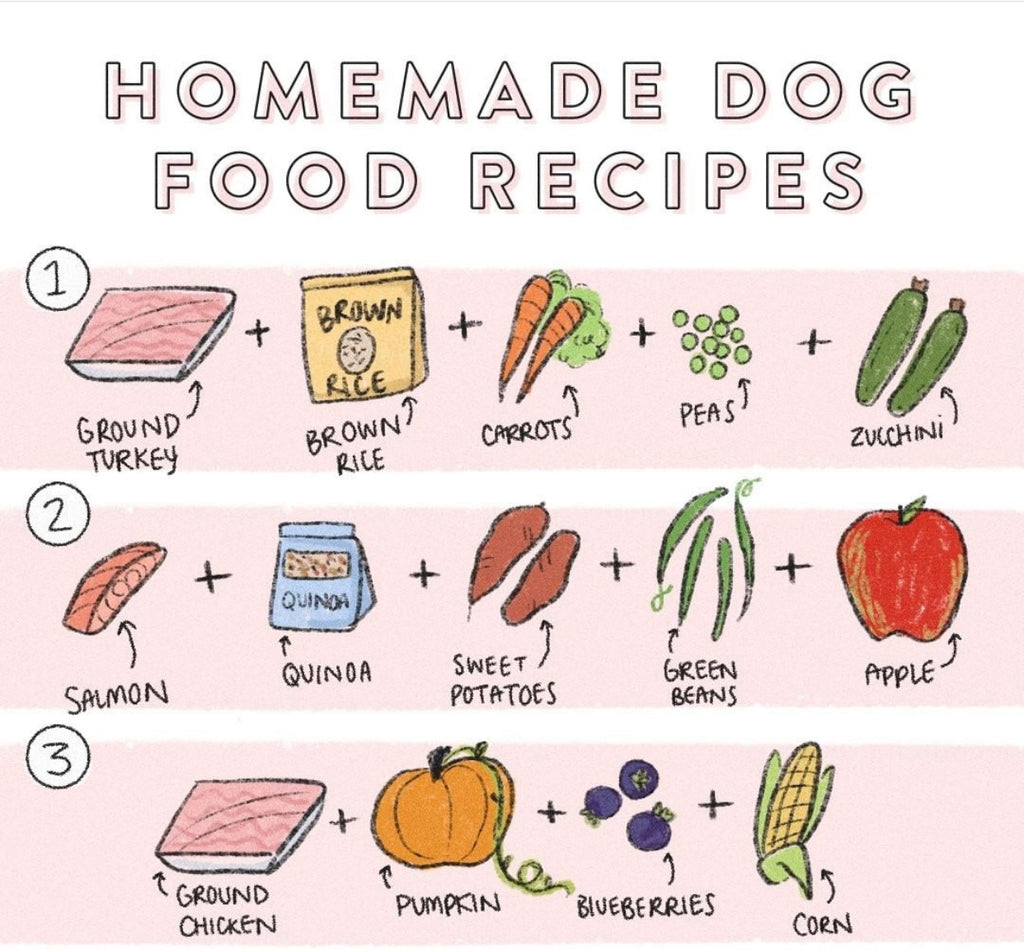The image is a neatly designed chart titled "Homemade Dog Food Recipes" in large, hollow, pink letters at the top. The chart is organized into three rows, each displaying a different recipe. 

The first row features a hand-drawn, colored picture of ground turkey, a bag of brown rice, two carrots, peas, and zucchini, with each item's name labeled in black capital letters beneath the drawings. Thin, curved arrows point from each label to its corresponding illustration, making it easy to identify each ingredient.

The second row presents a recipe consisting of salmon, quinoa, sweet potatoes, green beans, and an apple. Again, each ingredient is represented by charming hand-drawn images and labeled similarly, with arrows connecting the labels to the drawings.

The third row showcases a combination of ground chicken, pumpkin, blueberries, and corn, following the same visual style with labels and connecting arrows.

The entire chart maintains a cohesive, light pink background, making it visually appealing and simple to follow for anyone looking to prepare homemade dog food.